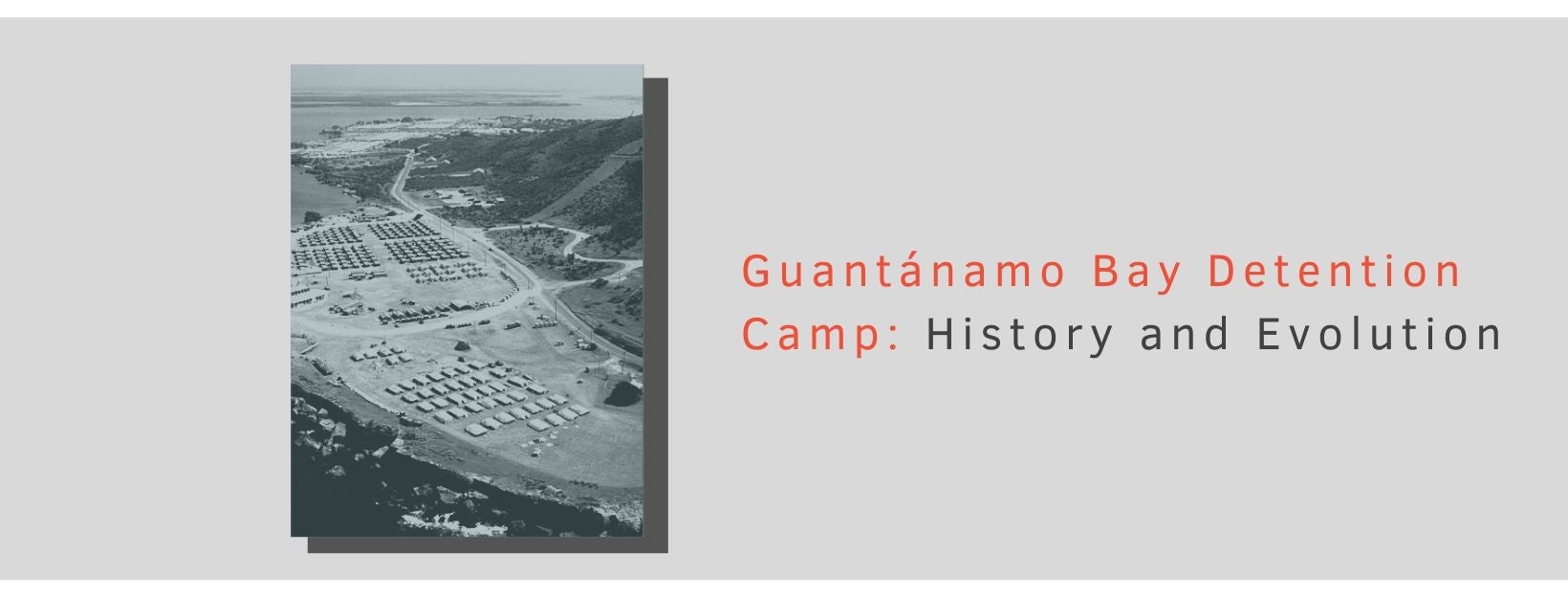The image is a detailed, long horizontal rectangle with a light gray background. On the left side of the image is a black and white aerial photograph depicting the Guantanamo Bay Detention Camp. This photograph, which appears digitally affixed to a wall, shows a sprawling encampment nestled amongst hills with the ocean faintly visible in the background. The camp comprises numerous rows and columns of small, square structures that could either be tents or buildings, hinting at its capacity to hold a large number of individuals. The perspective of the shot suggests it was taken from an elevated position, likely an airplane or helicopter, providing a comprehensive view of the layout and surrounding topography.

On the right side of the image, there is text in a distinguishable format: in orange, it reads "Guantanamo Bay Detention Camp:" followed by "History and Evolution" in black. This text likely indicates the title of the book or the section of a website dedicated to educating viewers about the history and development of the controversial detention facility.